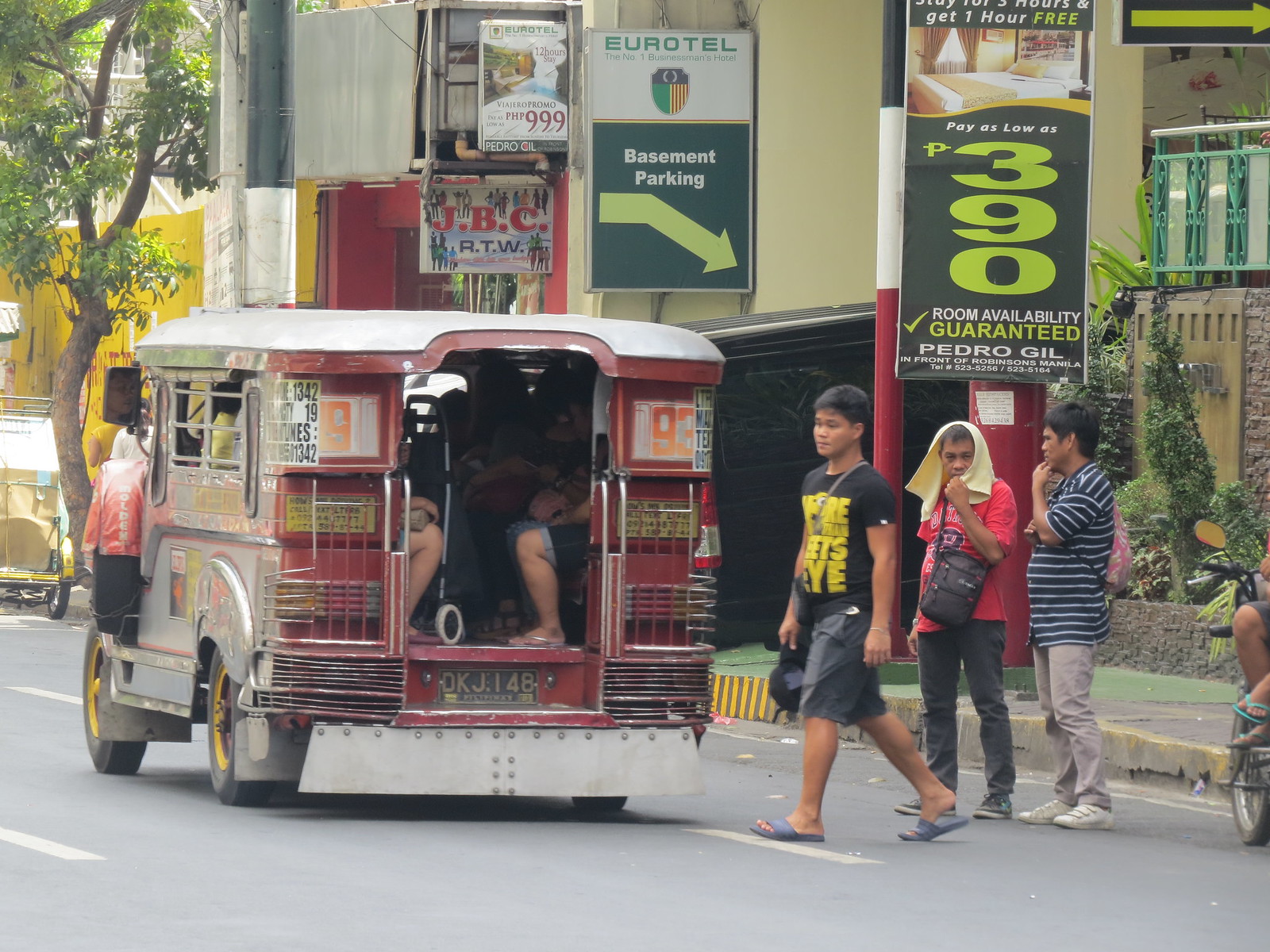In this bustling city street, likely located in Asia or Southeast Asia due to the appearance of the people and the signage, a red open-ended shuttle bus is prominently featured on a gray road marked with white dashed lines. The bus, with silver accents and signage, allows easy access for passengers through its open back. Nearby, three men are visible crossing the street: one in a black shirt and gray shorts, another in a red t-shirt and gray pants, and a third in a gray and white striped shirt with khaki pants. Surrounding the scene are various signs indicating services and promotions, such as "JVC RTW," "Basin Parking," mentions of "Pedro Gil in front of Robinson's Manila," and details like "Room Availability Guaranteed" and "Pay as low as 3.90." Lush greenery with brown trunks and green foliage frames the urban setting, adding a touch of nature to the vibrant cityscape.